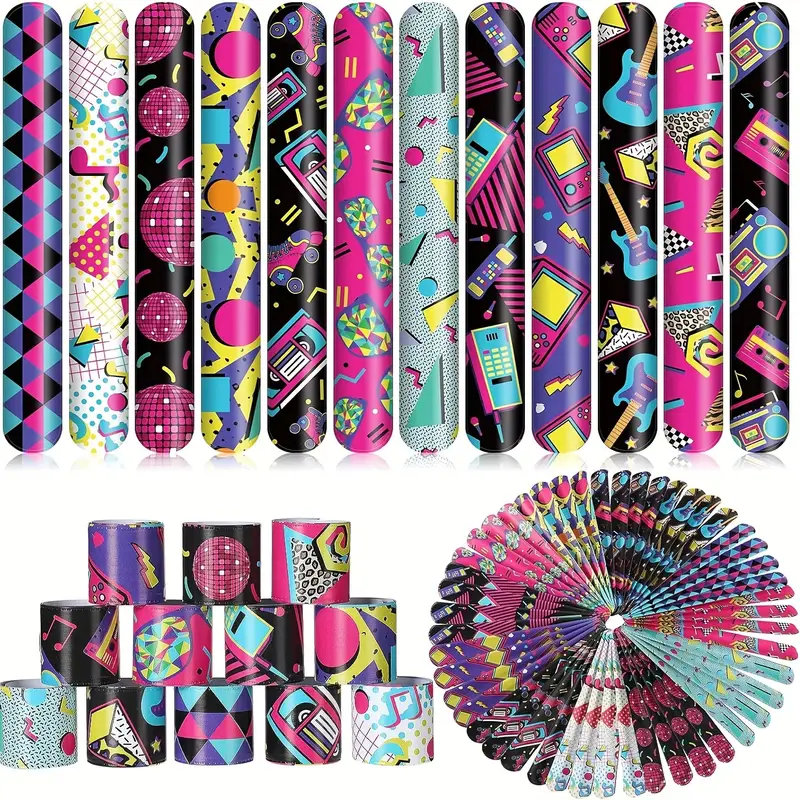The image vividly showcases a large collection of slap bracelets with vibrant and varied designs. The top portion features 12 slap bracelets arranged vertically side by side, each adorned with extremely busy, colorful patterns such as black backgrounds with guitars, diamonds checkered in purple and pink, alternating black and blue, and more. Below this lineup, a tower-like stack is constructed from rolled-up slap bracelets—five at the base, topped with four, then three more. To the right of this tower, a striking pinwheel-like circular formation of approximately 50 to 60 slap bracelets radiates outward, with an empty space in the center. The diverse array of designs includes diamond shapes, music notes, disco balls, cassette boom boxes, sunglasses, confetti, triangles, cell phones, Gameboys, Walkmans, guitars, cheetah print, and more, giving the overall arrangement a fun, flirty, and feminine feel.